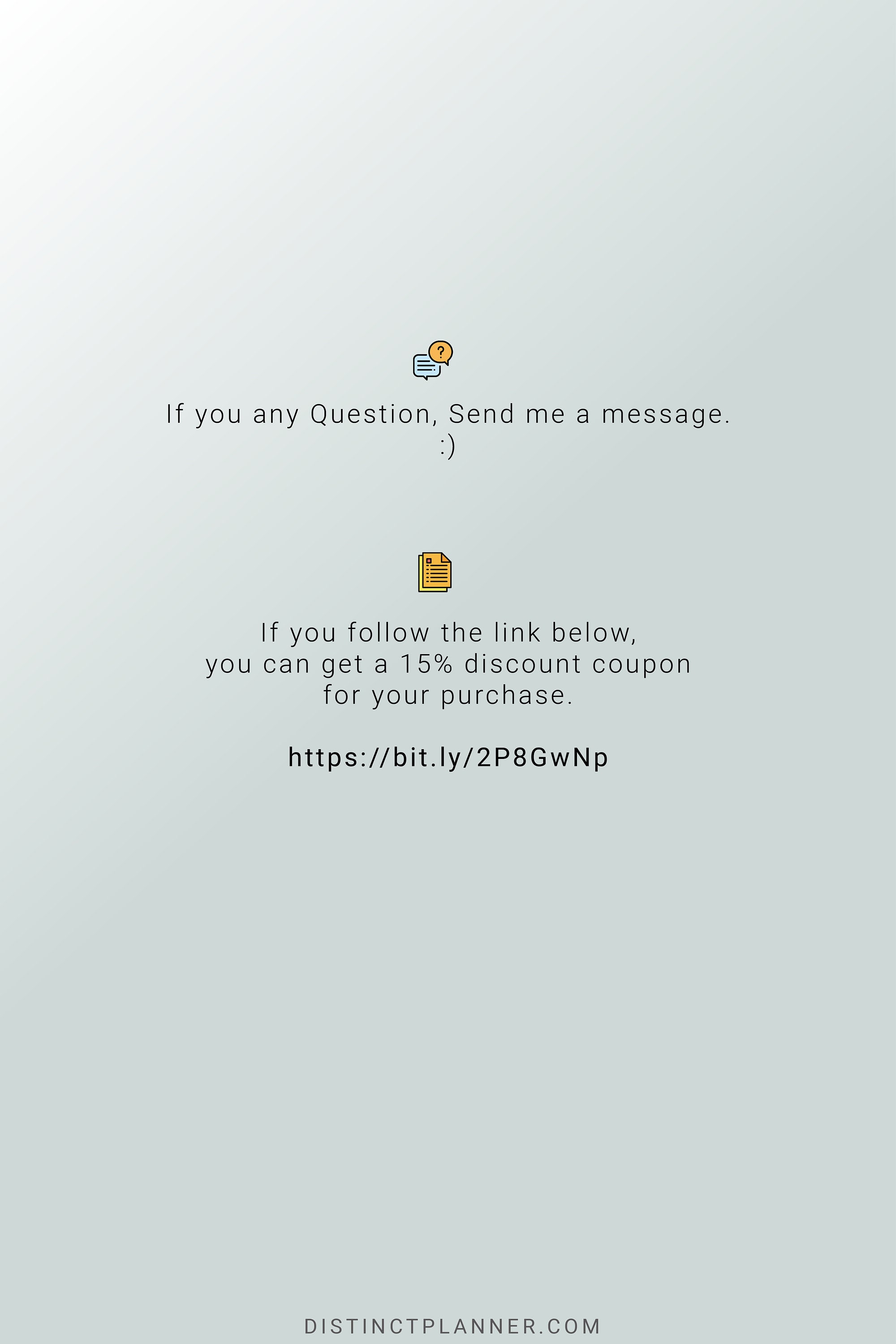The image is predominantly gray, featuring text and emojis as part of a screenshot from a website. At the bottom, there is a web address that reads "distinctplanner.com." 

Toward the top, approximately a third of the way down, there is an emoji of a message box with a question mark, accompanied by the text, "If any questions, send me a message. :)". However, there is a typo, as the phrase should read, "If you have any questions, send me a message." Additionally, the sentence contains a comma splice due to the capitalization of "send."

Below this, there is an emoji resembling a yellow document with a red dot in the upper left corner. This document emoji is followed by the text, "If you follow the link below, you can get a 15% discount code for your purchase." There are no typos in this section.

Afterward, a short URL is provided, which is: "https://bit.ly/2P8Gwnp". The capitalization is also specified as "2 capital P 8 capital G lowercase w uppercase N lowercase p."

Overall, the image is a screenshot of a promotional website displaying information about how to receive a discount code by following the provided link.